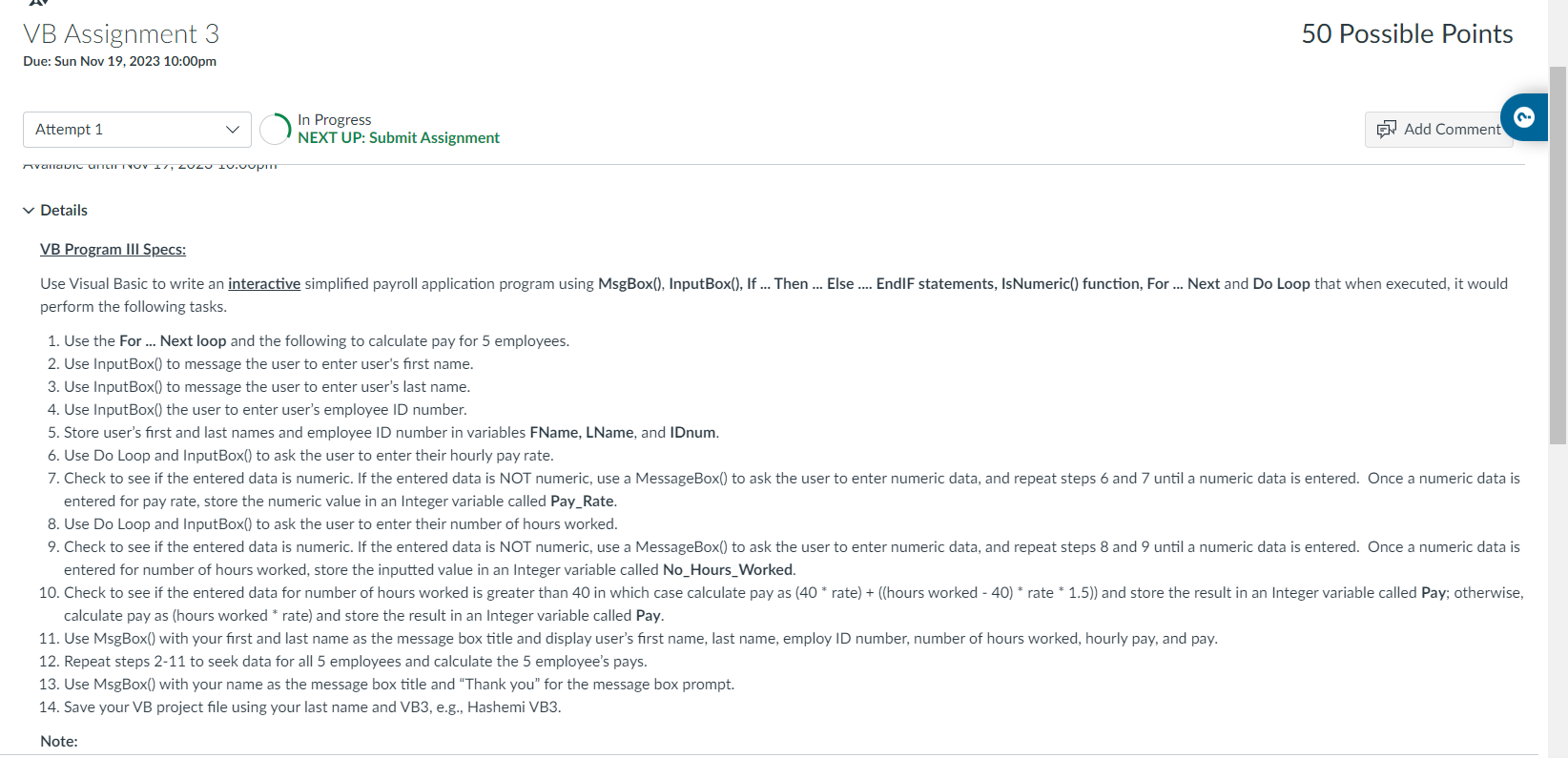The image depicts a computer screen displaying the title "BB Assignment 3." Below the title, there's a section labeled "Details" that lists several cryptic instructions related to a programming task. The task appears to involve creating an interactive, simplified payroll application using Visual Basic. The instructions specify the use of various programming constructs such as "If-Then loops," "For-Next loops," "Do loops," and the "InputBox function" to interact with the user. Furthermore, it mentions saving the project file using the format "lastname_VB3." The background of the screen is white, and the text is black. This appears to be a homework assignment, likely for a computer science course, provided through a learning platform.